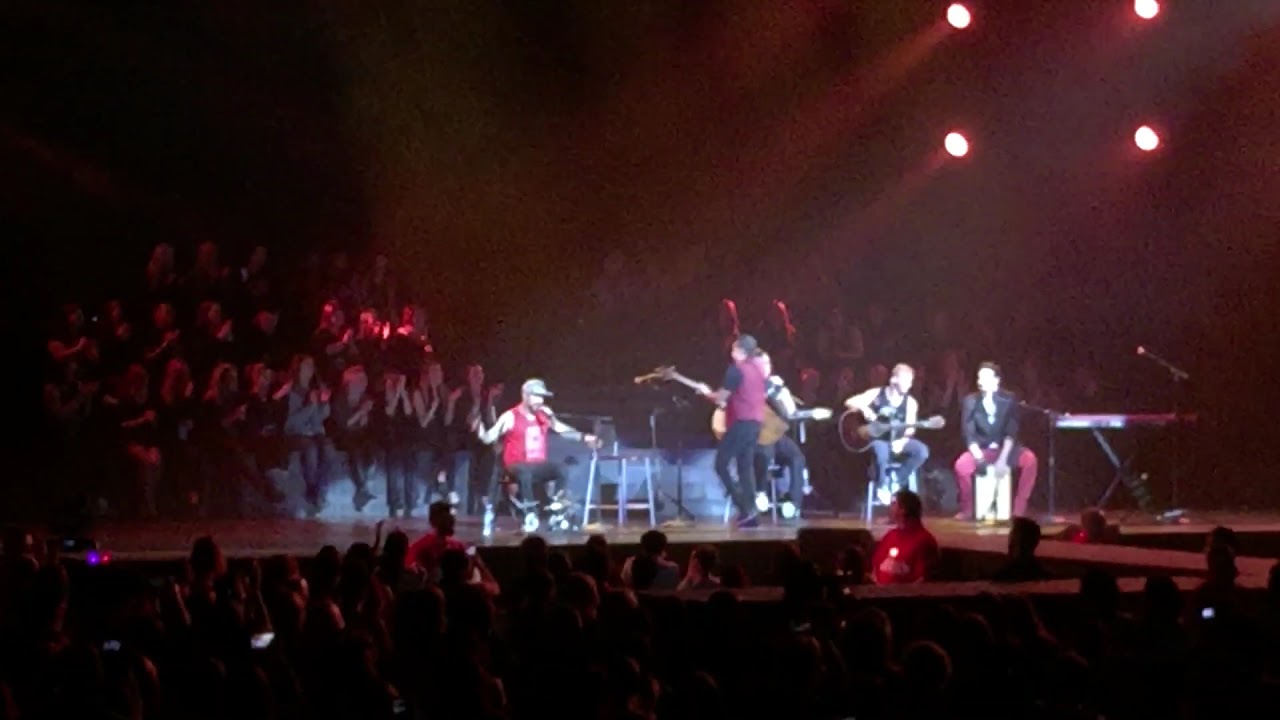In this image of a dimly lit, indoor concert environment, a rectangular stage with a narrower extension in the center is surrounded by an audience of over 100 people, capturing the performance on their phones. Positioned in the middle of the image, five musicians are arranged across the stage. On the far right, one performer in red pants sits on a white seat beside a piano, singing into a microphone. To his left, another musician plays the guitar, followed by a third individual playing an electric bass. To the left of the bass player, a fourth musician in a red shirt plays an acoustic guitar, and next to him, another person in a red tank top with a baseball hat holds up an object in his right hand while speaking into a microphone. Overhead, stage lights cast a mix of red, black, white, gray, maroon, purple, and pink hues, giving the performance a vibrant yet intimate atmosphere.